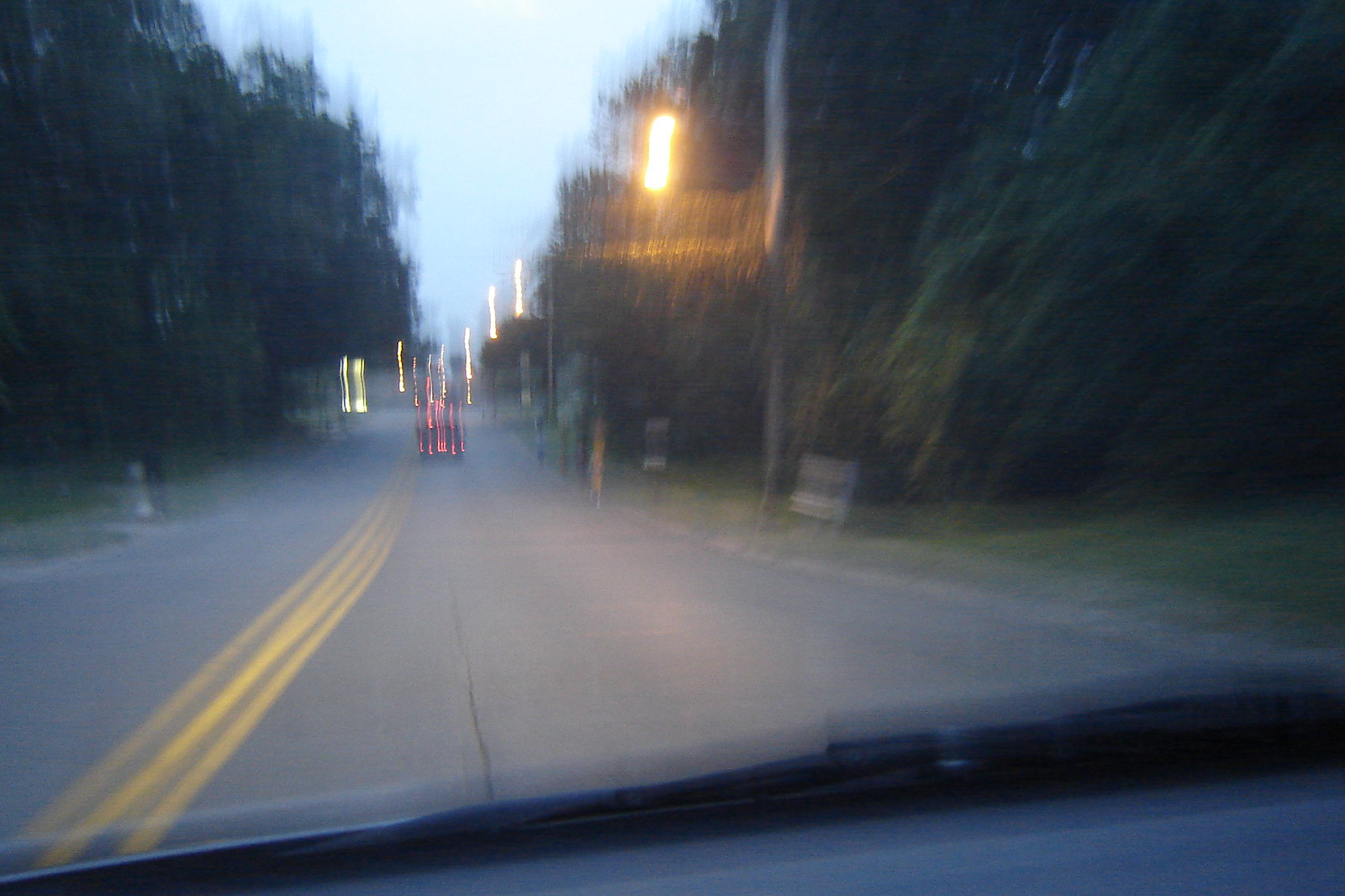A blurred photograph captures a road scene taken from a moving automobile. In the image, out-of-focus streetlights cast a hazy glow, while the distant taillights of a vehicle create streaks of red light. The yellow lines that typically divide the lanes appear wavy and duplicated due to the motion blur. Surrounding the roadway, dense greenery and trees form a soft, indistinct backdrop to the scene.